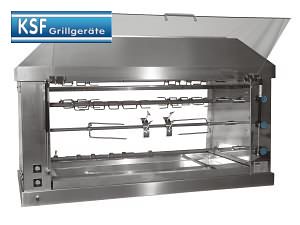This image is a color photograph displaying a stainless steel, industrial-grade rotisserie grill against a white background. The top left corner features the company logo, a blue rectangle with white stripes along the top and bottom, and the text "KSF Grill Geräte" in white lettering. The grill itself is encased in a sleek, reflective silver housing with a slanted roof-like top. The front of the grill has a hinged, see-through glass door that is currently open, exposing the interior.

Inside the grill, there are several horizontal rods. The middle rod is equipped with two large fork-like prongs designed for securing poultry or lamb as it rotates during cooking. Additional rods with chain links and skewers occupy the upper and lower sections, intended for various grilling applications such as roasting hot dogs or other items. 

On the left side of the grill, there are two black squares featuring silver circles that might be buttons or indicators. To the right, there are three blue circular knobs, likely controls for the appliance. The entire setup is polished and professional, emphasizing the high-quality construction of the cooking device.